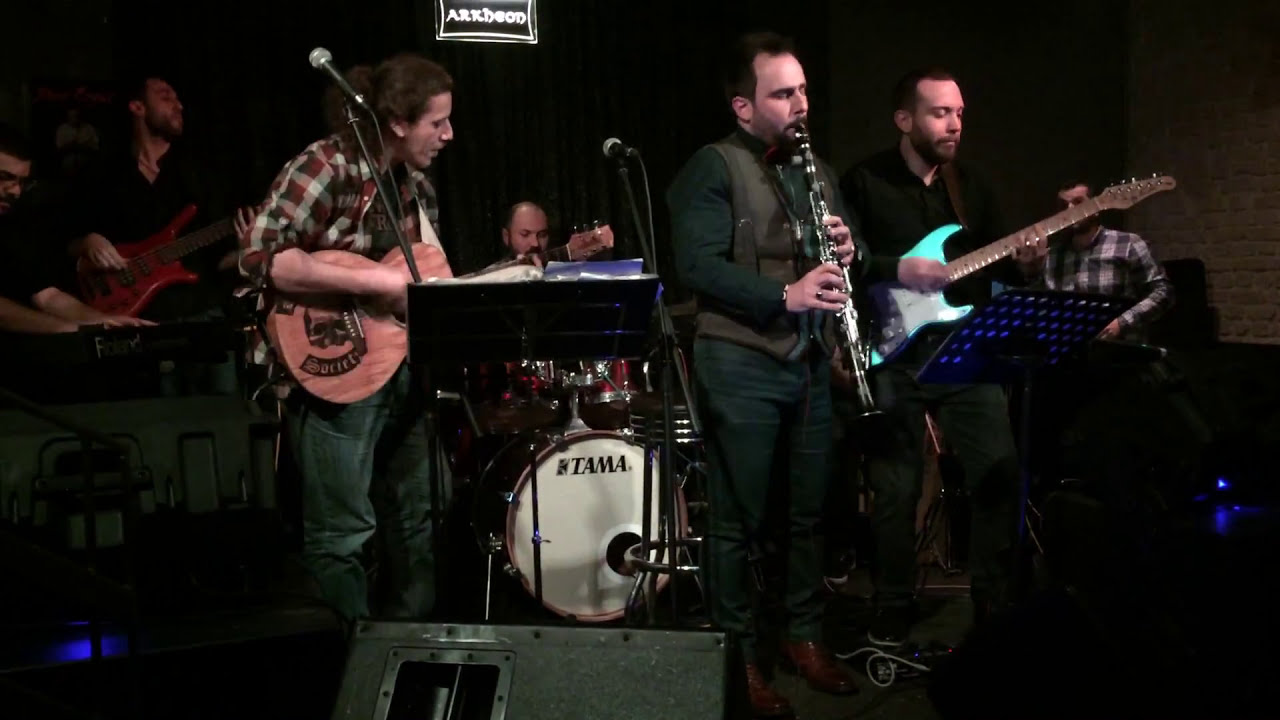The photograph captures a band of six musicians performing on a stage inside a building with a dark background. From left to right: the first man, dressed in green, plays a brass instrument, possibly a clarinet. Next to him, another man with his hair pulled back in a ponytail wears a red and white striped shirt while playing a guitar, which has a distinctive greenish-blue and white color. Further to the right, a bearded man plays an acoustic guitar. Behind them, a drummer sits at a drum set with "Stama" or a similar name in black letters on the white drumhead. The far-right features a man whose instrument is not clearly visible. Also present is a man at an organ. Above the stage, there's a sign that says either "Art Neon" or "Arc Beam," hinting at the possible band or venue name.